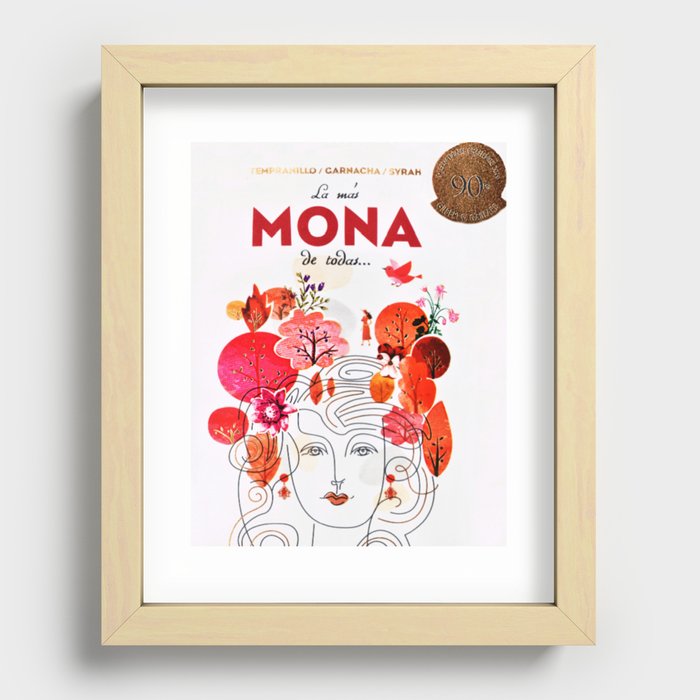The image is of a poster framed in light brown wood, hanging on a light blue wall. The background of the poster is white, with a light blue border about an inch in from the frame. In the top right corner of the poster, there is a gold round object with the number "90" in black on it. At the top left of the poster, gold lettering spells out "Carmaca Syrian," followed by black lettering that reads "La Mas." In large, bold red letters, it says "Mona." Below that, it states "De Tadis" in cursive-like black font. 

The central image is a detailed black-and-white sketch of a woman's face with flowing, wavy hair accentuated by zigzag and wiggly lines. Her lips are strikingly red, and she wears red earrings in each ear. Surrounding her head are patterns of orange and pink leaves, and small circles, contributing to the decorative flair of the image.